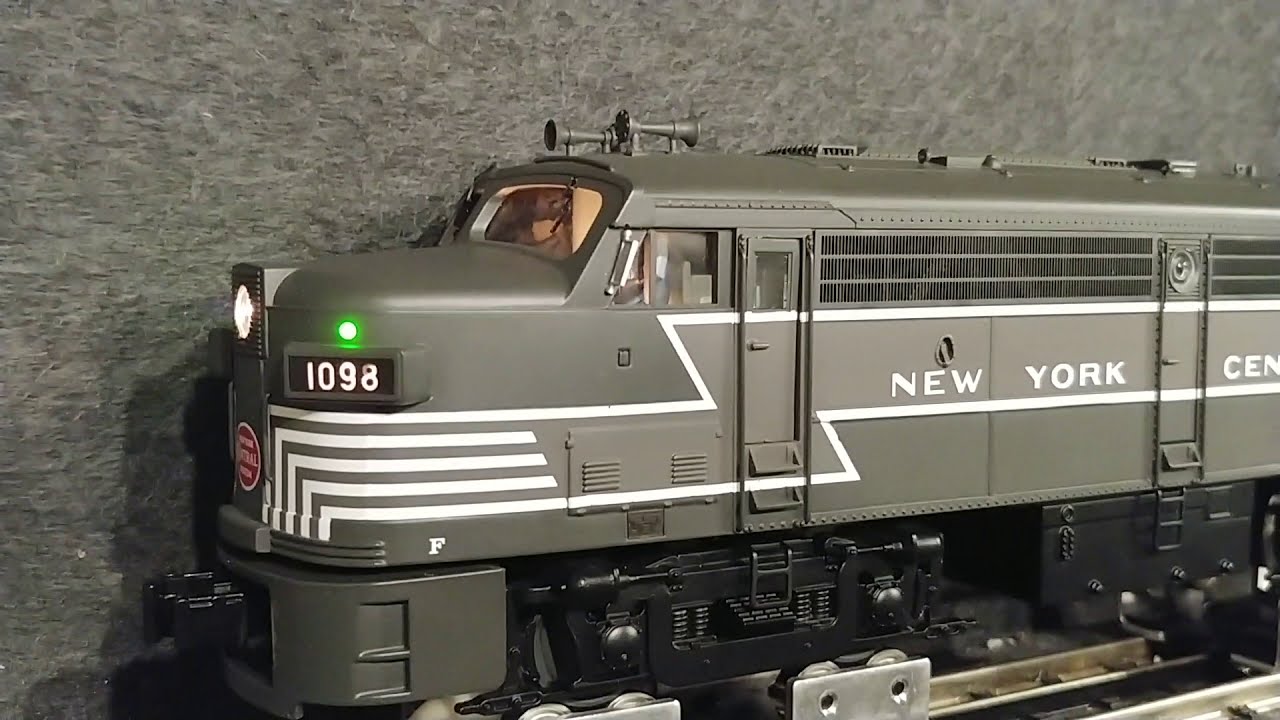This photograph features a detailed model train engine set against a textured dark gray background, evocative of painted wood. The model appears meticulously crafted, with the train painted in a deep gray-green hue. Prominently displayed on the front left of the train is the number 1098, situated below a circular lime green light angled slightly. Above this, a bright white headlight is noticeable, adding an authentic touch to the miniature locomotive.

The side of the train is adorned with multiple white stripes and the partially visible text "New York CEN," likely an abbreviation for New York Central, printed in bold white capital letters. Atop the cab of the train, two horns are visible, contributing to the realism of the model. The intricacies extend to the cabin's interior light and the black wheel fixtures, which contrast elegantly against the lighter silver or brass-colored rails beneath.

The model train's orientation suggests a left-facing direction, inviting viewers to appreciate the finely detailed craftsmanship, from its exterior paint to the precise lettering. The setting appears to be indoors, with the backdrop and display suggesting a deliberate, controlled environment designed to highlight the features of this impressive model train.